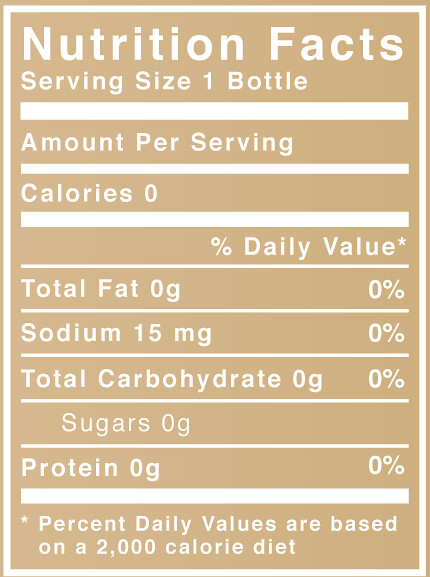This is an image of a Nutrition Facts label, typically found on food items. The label features a tan background with white lettering and a brown outer border with a white inner border. The text reads "Nutrition Facts" in bold white letters at the top. Below that, it states "Serving Size 1 bottle" with a white rectangle underline, followed by "Amount Per Serving" in a smaller white rectangle outline. It indicates "Calories 0" with a medium-sized white rectangular outline. The label then lists the "Percent Daily Value," underlined by a white line, followed by detailed nutritional information: "Total Fat 0 grams, 0 percent" with an underline; "Sodium 15 milligrams, 0 percent" with an underline; "Total Carbohydrate 0 grams, 0 percent" with an underline; "Sugars 0 grams" with an underline; and "Protein 0 grams, 0 percent" with a large white rectangular underline. At the bottom, there is a star indicating that "Percent Daily Values are based on a 2,000 calorie diet."